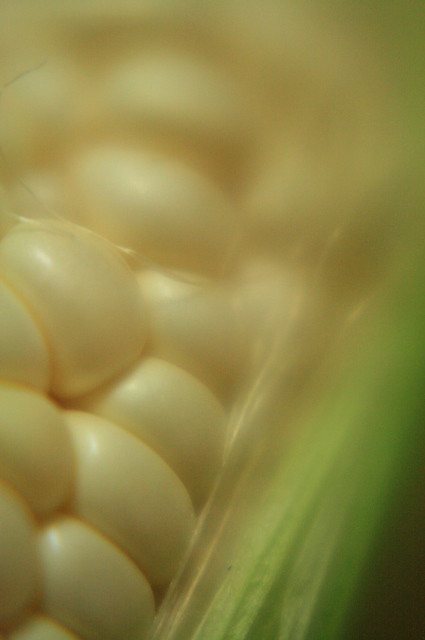This image showcases an ultra close-up of an ear of corn, highlighting numerous corn kernels in vivid detail. The kernels appear pale, light, whitish-yellow, gleaming as they catch the light. The husk, still partially enveloping the cob, ranges from deep green to lighter, beige shades and has peeled back to expose the kernels. Threads from the husk drape across the corn, adding texture. The top of the photo has a diffused, hazy quality, softening the view of the kernels, while the bottom features a black hazy area. The kernels themselves are arranged in a curved pattern reminiscent of teeth, showcasing both their yellow edges and the white gleaming tips where the light hits them.